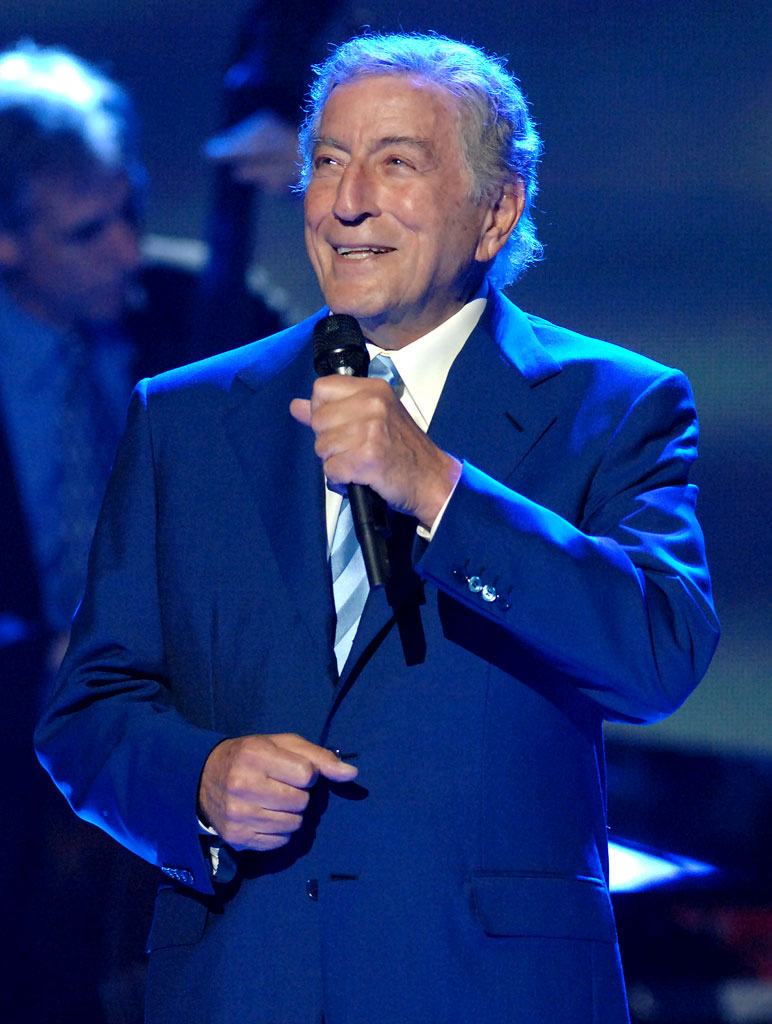An older man, likely in his 60s or 70s, is standing on a stage, smiling and holding a black, shiny microphone in his right hand. He is dressed in a dark blue suit paired with a white button-down shirt and a striped tie featuring shades of blue and light blue. His medium-length, gray hair appears bright blue under the illuminating stage lights. Off to his left, in the blurred background, another man is seated, seemingly playing a stringed instrument, which could be a bass guitar or a cello. This background figure is also donning a suit. The stage lighting casts a bluish hue over the entire scene, adding a vibrant glow to both men's attire and the foreground subject's hair. The overall ambiance is one of a lively musical performance.